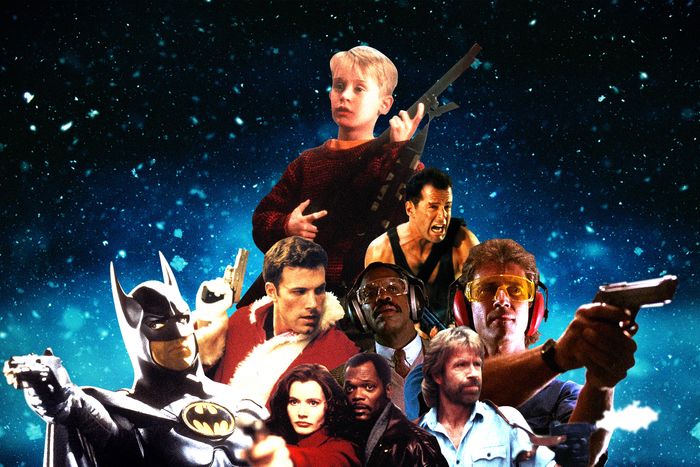The image portrays a dramatic space setting with a dark black-to-blue gradient background and star-like white flecks scattered across. Prominent film characters are collaged in a triangular formation. At the pinnacle stands Kevin McAllister, portrayed by a youthful Macaulay Culkin from "Home Alone," donned in his iconic red sweater, holding a BB gun rifle. Descending slightly right is Bruce Willis as John McClane from "Die Hard," with his receding hair and a pained, screaming expression. To the left, Ben Affleck’s clean-shaven face, garbed in a Santa Claus costume, aims a gun.

Below McClane, Danny Glover, and Mel Gibson embodying their "Lethal Weapon" characters. Glover wears black earmuffs and clear goggles, while Gibson has yellow goggles and red earmuffs, both in blue shirts and armed. Nearby, Chuck Norris, recognizable by his beard and a holster, is poised with a gun.

Further down, Samuel L. Jackson in a leather jacket and gray scarf stands beside Geena Davis in a red coat, representing "The Long Kiss Goodnight." Batman, stoically holding a gun with the iconic yellow and black bat symbol, is positioned on the lower left, preparing to confront a clown villain. All characters are referencing their notable Christmas-themed films, enhancing the image's festive, snowy ambiance in a galactic backdrop.